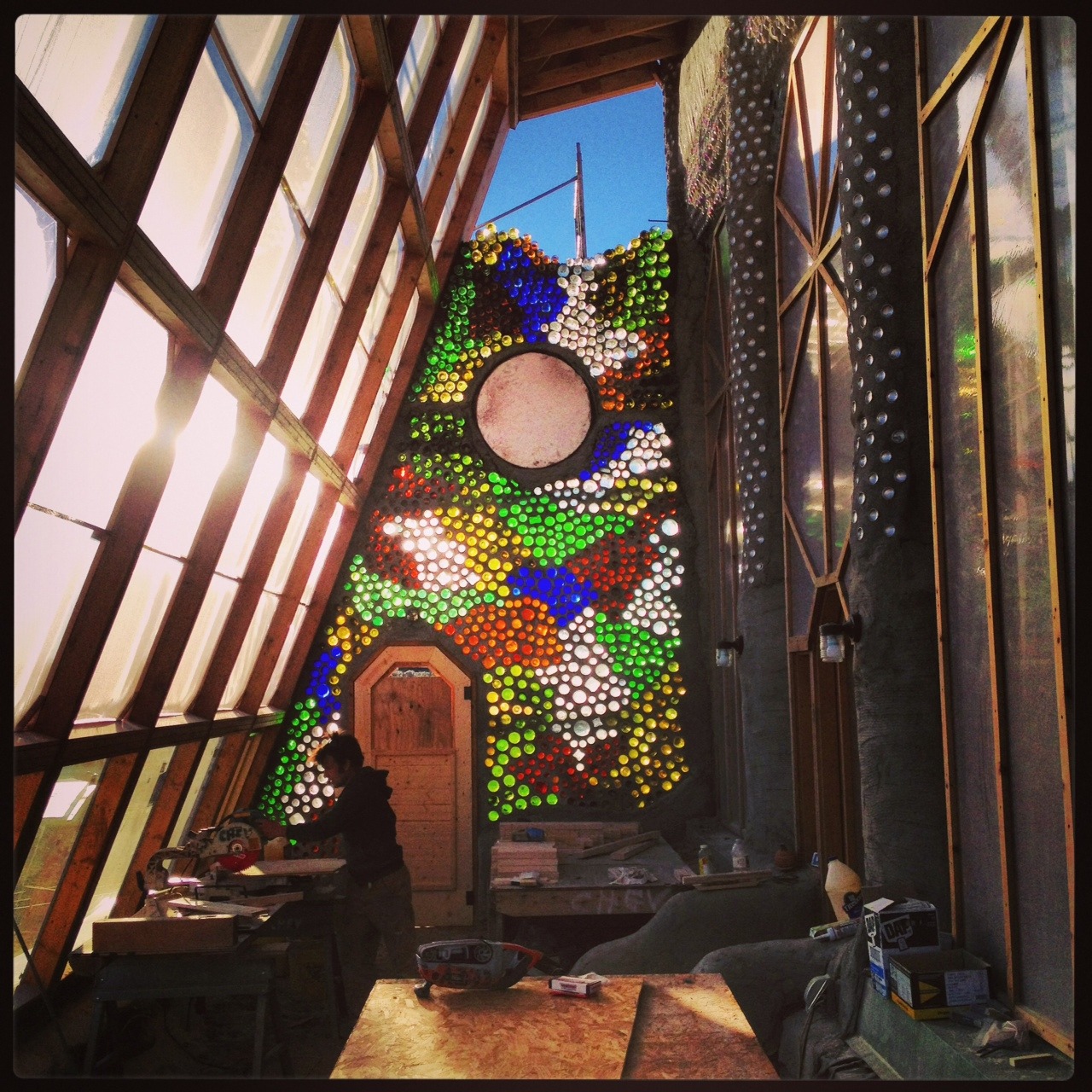In this detailed scene, the room appears to be a rustic workspace, possibly part of a church or an artist's studio. It features one wall with a colorful, almost mosaic-like stained glass window that comprises various colors such as orange, green, white, red, yellow, and blue. This vivid window allows some natural light into the room but is centered behind a large, sturdy wooden door. On the left-hand side, the wall and ceiling form an A-frame with a series of windows that are divided by wooden planks, letting in ample light. The right side of the room is darker, with two lamps fixed on the wall, providing additional illumination.

A man, likely Caucasian with brown hair, dressed in a dark hoodie and khaki pants, is positioned near the bottom of the scene, bent over a table. He appears to be woodworking, using a table saw, surrounded by various tools and pieces of wood scattered around. This workshop setting is cluttered with multiple tables, saws, and additional woodworking tools. Near the camera, there's another table featuring a different tool, perhaps another type of saw. The space exudes a rustic vibe, enhanced by the wooden elements and the artisanal feel of the colorful stained-glass window.